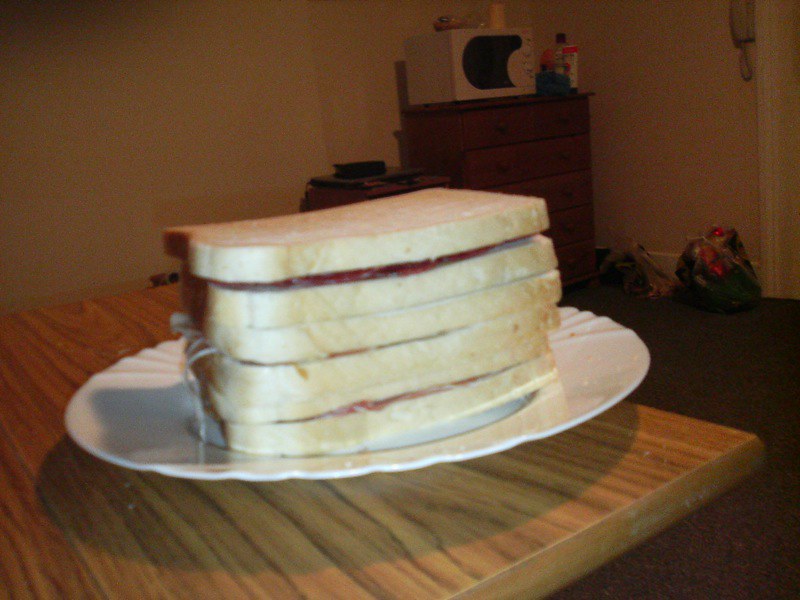In a dimly lit room, this photo captures a wooden table with a dark wood grain and a white porcelain plate at the forefront. On the plate, there's a towering sandwich made of six pieces of white bread with an indiscernible red filling and possibly some strings of lettuce peeking out from the left side. The shadow of the plate falls across the table, adding to the image's subdued ambiance. The background features a beige or cream-colored wall, a dresser with a white microwave on top, and various indistinguishable items scattered about. The floor appears to be carpeted, though its color is obscure due to poor lighting. Additionally, a landline phone is mounted on the wall to the right of the dresser, and bags of items are visible on the floor nearby.